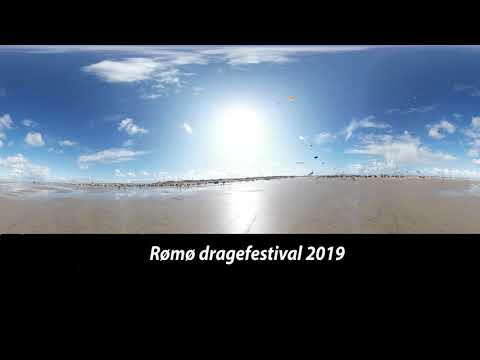The image captures a bustling beach scene likely taken during the Romo Draga Festival 2019, as denoted by the white text on a black background at the bottom of the image. The photo is wide but cropped at the top and bottom, with a thin black bar at the top and a larger black bar at the bottom, providing a panoramic yet low-quality view. The beach is shown under a clear, deep blue sky with a few wispy clouds, and a bright sun near the center casts a streak of light across the wet, shiny sand, suggesting a late afternoon setting. The sand is a light tan, and there are scattered people throughout the scene, possibly some birds on the right-hand side, although the picture’s blurriness makes it difficult to discern precise details.